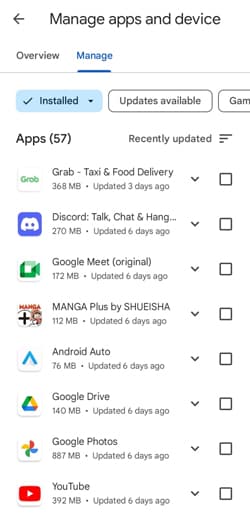This screenshot features a detailed interface with a white background, primarily situated in the upper left-hand corner. At the top, a gray left-pointing arrow is displayed, followed by the text "Manage Apps and Device" in gray. Three lines below this on the left, the word "Overview" appears in gray. To the right, "Manage" is highlighted in blue with a blue underline. A light gray horizontal line separates these elements from the content below.

Beneath the separator, there are several buttons. To the left, a button stands out with a blue background featuring a black checkmark on its left and the text "Install". This button is accompanied by a drop-down arrow. Next to it, a button with a white background outlined in gray bears the text "Updates Available" in gray. Only the beginning of the third button is visible, showing the text "GAM".

Approximately two lines down on the left side, the term "Apps" is displayed in bolded black, followed by the number 57 in parentheses. On the right side, the phrase "Recently Updated" appears in gray, accompanied by three horizontal lines, each shorter than the one above.

Below, a list is presented with icons on the left, the names of the apps next to the icons, a drop-down arrow beside each name, and a checkbox to the right of the arrow. The first app listed is "Grab, Taxi and Food Delivery", followed by "Discord, Talk, Chat and Hang", "Google Meet (Original)", "Manga Plus by SHUEISHA", "Android Auto", "Google Drive", "Google Photos", and "YouTube".